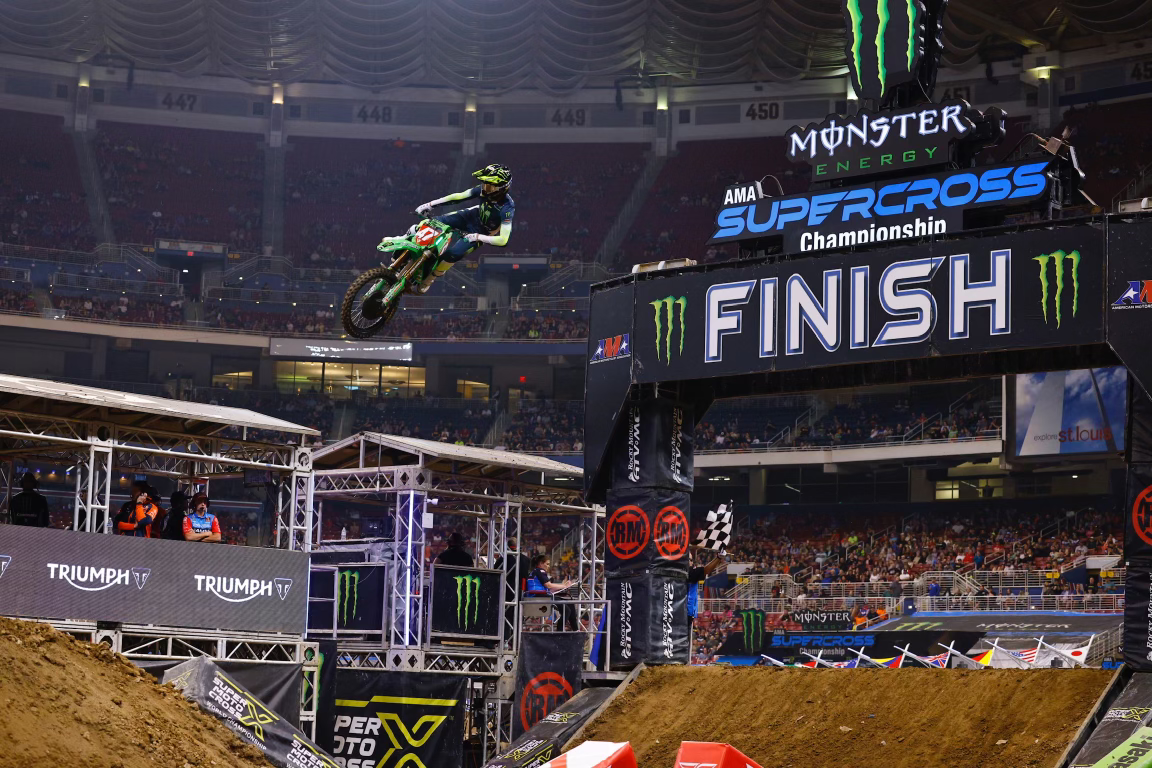This photo captures an exhilarating moment during a Monster Energy AMA Supercross Championship event inside a large stadium. Center stage, a rider on a green dirt bike, donned in a blue shirt and blue pants, with a striking black, yellow, and green helmet, is captured mid-air, twisted almost completely sideways. Below him, the dirt ramps and the bustling crowd frame the action, highlighting the dynamic atmosphere. To the right, two stations are set up; one featuring two people in orange shirts under a railing emblazoned with "TRIUMPH" in white letters, and another sponsored by Monster Energy, its distinctive green emblem prominently displayed. The stadium rows are marked with numbers 447, 448, 449, and 450, visible at the top. Dominating the right side of the image, a large black archway marks the finish line, adorned with the Monster Energy logo and the words "Monster Energy AMA Supercross Championship" in blue and "FINISH" in bold white letters beneath. This snapshot epitomizes the high-octane spirit of the event, emphasizing the skill of the stunt rider and the vibrant energy of the competition.